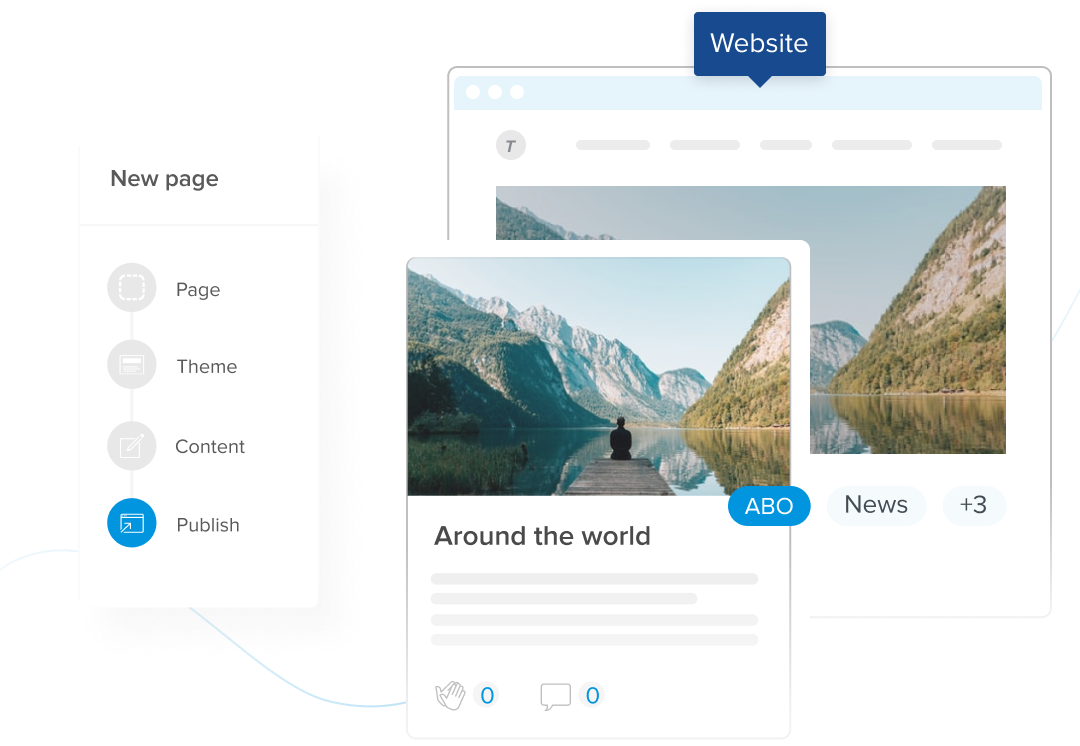**Detailed Caption for the Image:**

The image showcases a detailed mock-up of a web page. On the left side, a white rectangular section is labeled "New Page" in black text at the top, followed by a gray line. Below the line, there's a dark gray circle with a white square inside it. This section appears to be a sidebar menu.

On the right side of this menu, there are several icons and text areas, indicating different sections of the web page. The first icon is a page symbol with a gray circle and a white square inside it, labeled "Theme." The next section features a piece of paper with a pencil inside a dark gray circle and is labeled "Content." The final section is a dark blue rectangle with a web page icon and a white arrow pointing to it, labeled "Publish."

To the main content area on the right, there's a detailed mock-up of a website. This website mock-up features a main blue rectangular header that says "Website" in bold white text with a small downward-pointing arrow within it. The bezel of this mock-up includes three circles reminiscent of a Macintosh window controls. The main rectangle at the top is cyan blue. The background of the mock-up is white, showcasing five dark gray oval buttons, and a gray circle with a black "T" in the center.

Overlaid on top of this backdrop, though slightly obscured, is an image depicting a scenic view. This image consists of mountain ranges in the distance with gray and green hues. The nearest mountain, to the individual sitting at the edge of a dock, is dark green, covered with numerous trees. To the right of the person, another mountain is visible, gray in some areas but predominantly dark green due to foliage. The reflections of these mountains appear on the water in the foreground. The person, seen from behind, is wearing a black shirt and has brown hair.

Below this main scene, on the right-hand side, there’s a dark blue oval labeled "ABO" in white, with "Around the World" written boldly in black underneath it. Below this text are lines representing additional text, colored in dark gray. Additionally, there are icons resembling hands, representing clapping or celebration, with a blue "0" next to it, and a chat bubble also indicating a blue "0."

In the background section of the web page, there are more icons: a light blue oval labeled "News," and a circle with a plus symbol and the number three, "+3," displayed in black.